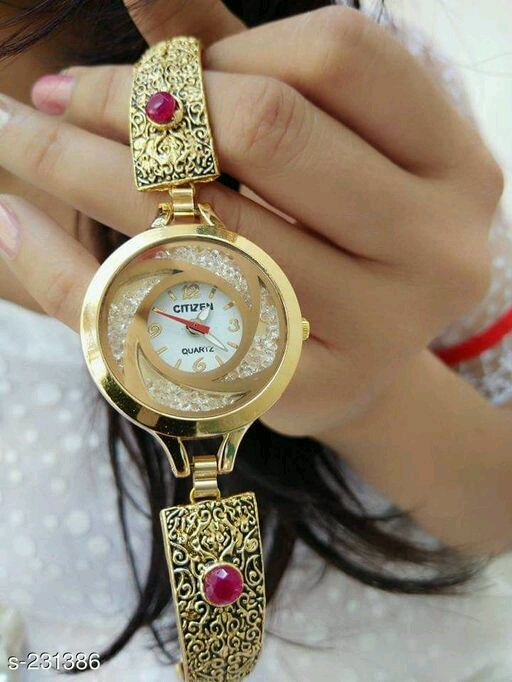In this detailed and vertical, rectangular image taken in real life, we see a person holding an elaborate Citizen watch with a predominantly gold design. The individual's nails are painted in a mix of red and white, and they appear to be wearing a white dress, their dark hair partially visible. The watch itself is ornate, featuring gold swirls creating a concentric circle design on the dial, and the bezel is thick, set with small crystals. The brand name "CITIZEN" is prominently displayed in black capital letters at the center, above the word "COURTS" in a smaller font over the number six. The time is shown with gold numerals for the hours 12, 3, 6, and 9, accompanied by gold lines for the remaining hour markings. The hands include a red second hand, a short white hour hand pointing at one, and a long white minute hand extending between four and five. The gold watch band is equally ornate, adorned with gold and black patterns and featuring small red gemstones, likely rubies, set on each section of the strap. The watch face indicates the time as 1:23 with the second hand positioned at the number ten. Hooks to a rectangular piece at the top and bottom, each garnished with a red gemstone encircled in gold, add to the timepiece's luxurious appeal. A segment of text "s-231386" is visible at the lower left corner of the image.